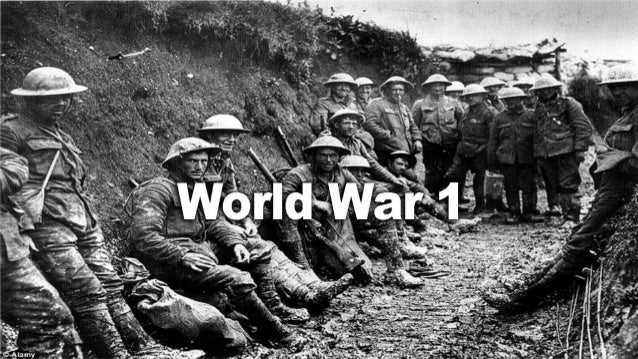This black-and-white photograph, with the text "World War I" superimposed in white at its center, depicts a group of approximately 16 haggard and worn-out soldiers. They are situated against a large dirt wall, which appears to be part of a trench, with some soldiers sitting or leaning on the left side and others standing towards the center and right. The rocky dirt pavement underlines the rough conditions they are enduring. Clad in disheveled military uniforms and rounded, wide-brimmed helmets, their dirt-smudged faces tell a story of exhaustion and prolonged battle. A few rifles casually rest against the trench wall, further emphasizing the wartime setting.